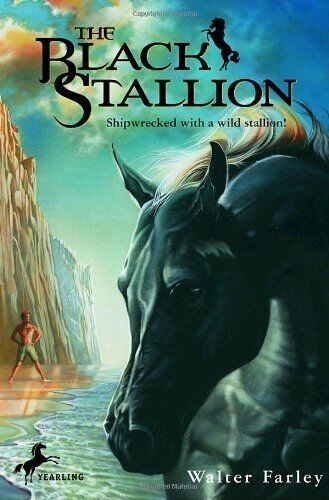This image is the cover of a book titled "The Black Stallion" by Walter Farley. The artwork is intricate and vividly portrays an outdoor setting during an early evening, suggesting a sunset with blue skies in the distance. The sky features some brownish clouds towards the left, blending into a vibrant horizon of orange and red hues. Below, there's a rugged cliff or mountain, and at the base of this cliff on the left-hand side, stands a man with no shirt, his arms on his hips. To the right of him, there is a body of water. Dominating the right side of the cover is a detailed, close-up image of a black stallion with a flowy brown mane, facing slightly left so the left side and part of the front of its head are visible. The title "The Black Stallion" is prominently displayed at the top of the cover in bold black letters with smaller text above it. Below the main title, in smaller black text, it says "Shipwrecked with a wild stallion." Additionally, there is an image of a horse rearing up on its hind legs to the right of the word "Black" in the title. In the bottom right-hand corner, the author’s name, Walter Farley, appears in white letters. The publisher's mark, "Yearling," is faintly visible at the bottom middle of the cover.